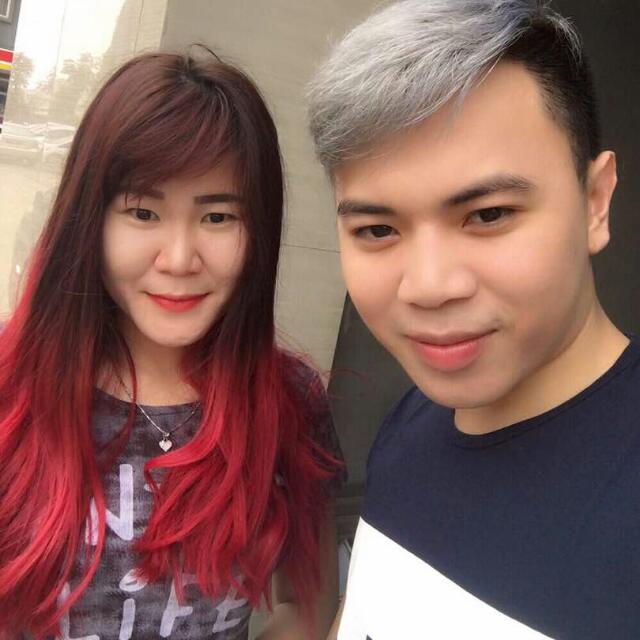The image captures a close-up selfie of two young Asian individuals standing side by side, with a subtle cityscape visible through a window behind them. On the left is a woman with long, dark hair that transitions to a bold red starting from around her shoulders to the tips, reaching down to her elbows. She is wearing a heart necklace and a shirt with an unclear inscription where only the word "life" is readable. Her makeup is minimal but noticeable, enhancing her healthy complexion. On the right is a man with a modern hairstyle featuring silver-dyed hair on the top, contrasting with his naturally dark hair on the sides. He's dressed in a blue t-shirt adorned with a white stripe across the chest. Both individuals are facing the camera directly and smiling slightly without showing their teeth. The background includes a part of a window with curtains, through which a few parked cars can be seen, suggesting an urban setting. The overall ambiance suggests an indoor environment with natural light filtering in from outside.